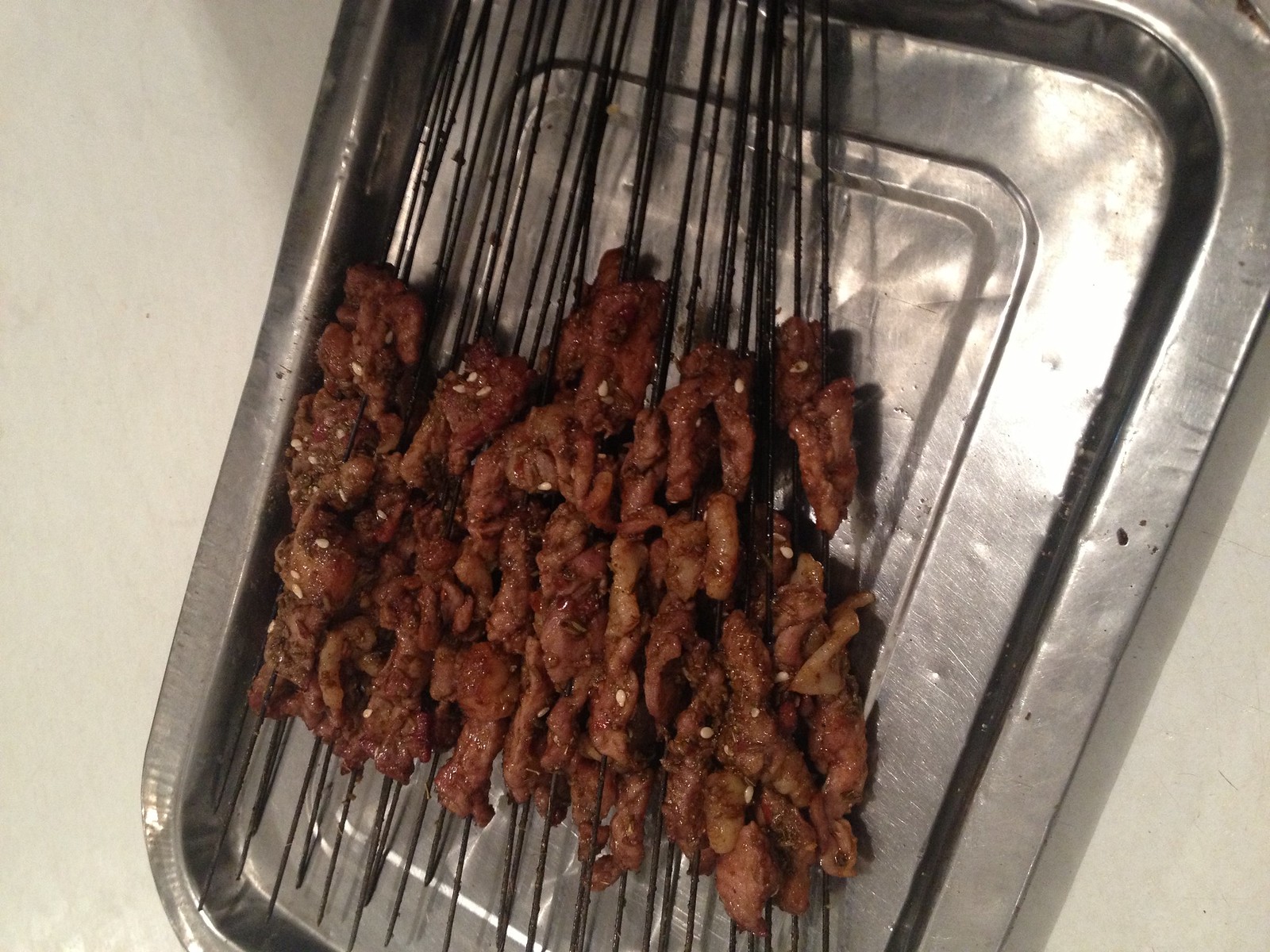In the image, a silver metal pan with a two-inch-deep lip, resembling an oven pan, rests on a flat white surface, possibly a table or countertop. The pan is filled with numerous skewers, potentially between 20 to 40, each threaded with pieces of brown meat, likely teriyaki chicken. The skewers, which are black, have a slightly charred appearance, indicating they were cooked over high heat, possibly on a barbecue. The meat glistens with a sauce and is generously sprinkled with white sesame seeds. A light source behind the camera creates a reflection on the stainless steel pan, enhancing the visual appeal of the scene.